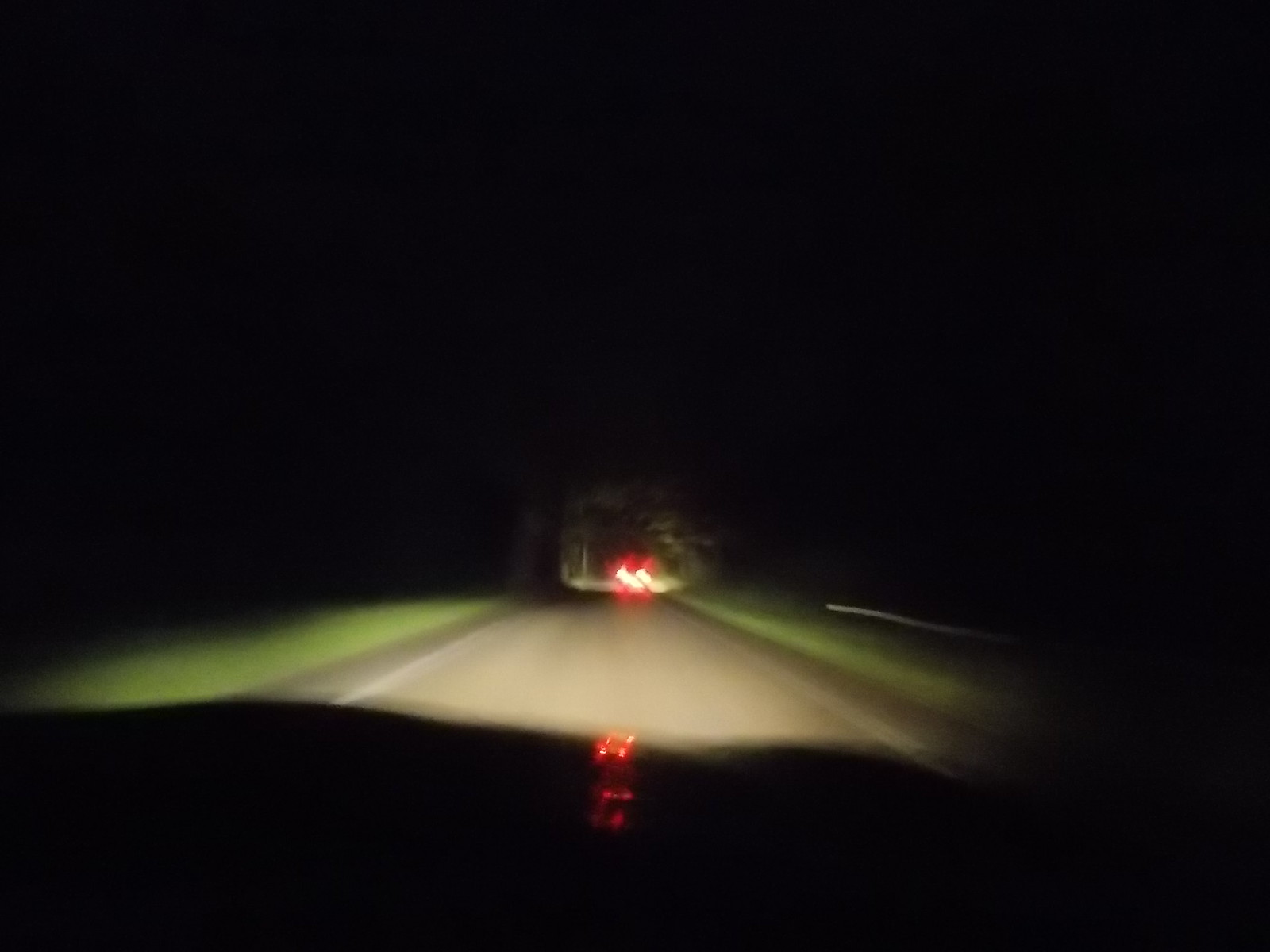This captivating image captures an outdoor night scene, viewed from inside a vehicle through its windshield. The sky is enveloped in a deep black, creating a dramatic backdrop. The black edge of the dashboard frames the bottom of the scene. Ahead, the vehicle's headlights illuminate a stretch of dark street, casting a pale gray hue on the asphalt. The street is bordered by patches of greenery on both sides, softly lit by the headlights. White lines run along either side of the road. In the distance, the red tail lights of another car are visible, their beams casting a glow on the road ahead and subtly illuminating the dashboard inside the viewer’s vehicle. On the right-hand side of the road, a small white line suggests the presence of a guardrail, adding an additional layer of detail to this nocturnal landscape.